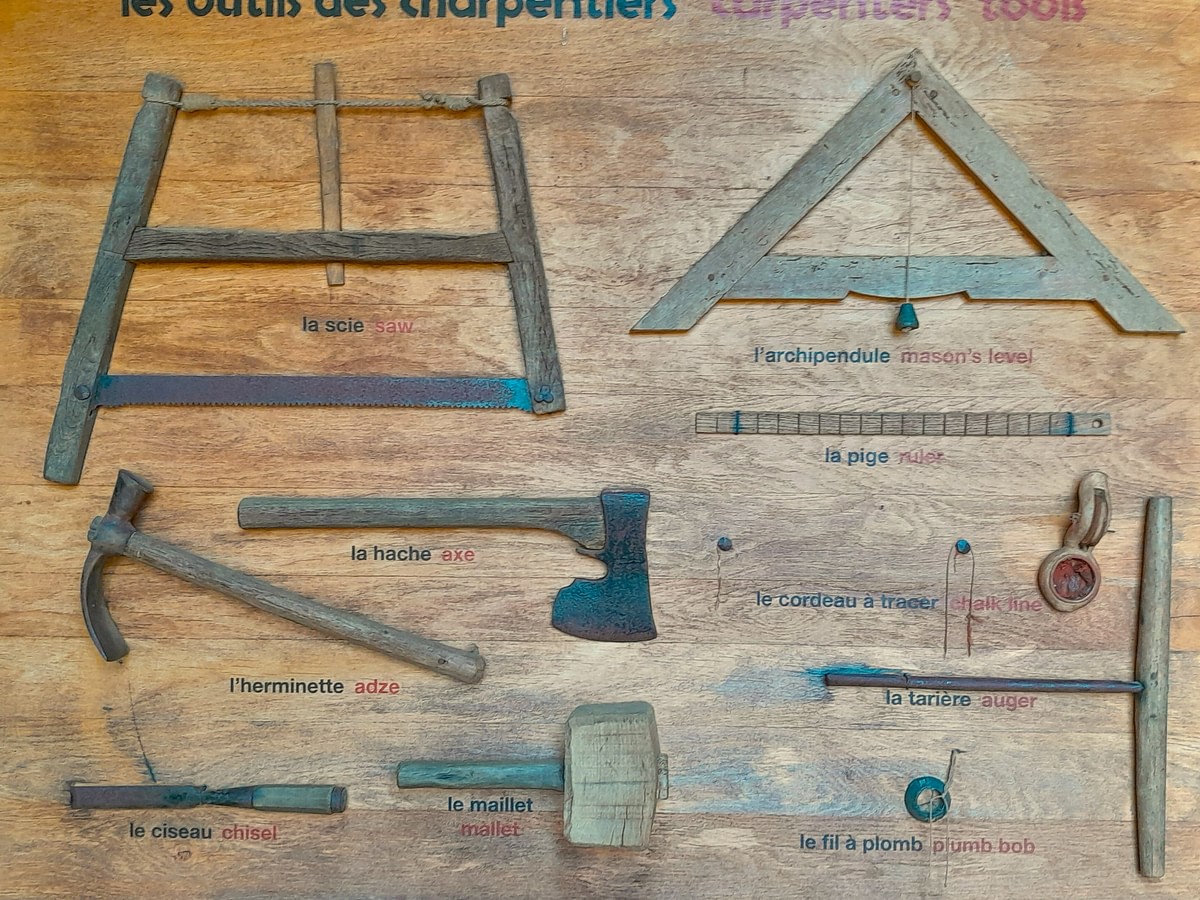The image depicts a collection of vintage carpenter's tools laid out on a wooden plank background. Dominating the center is an antiquated pull saw with a wooden frame and a rusted metal blade. Nearby, there is a primitive mason's level, consisting of a wooden body and a string ending in a bell-like plumb bob. A simple wooden ruler with drawn-in lines indicates old measuring techniques. A primitive auger, with its wooden handle and metal base, lies alongside a solid wooden mallet. A chisel with a wooden handle and a traditional vintage hammer are meticulously placed next to a vintage axe. The top of the image features text in French, followed by the label "Carpenter's Tools" in red, suggesting the historical significance of these items, possibly displayed in a museum setting. The tools have a robust and wide design, with the primitive measuring tools forming distinctive geometric shapes such as rhombuses and triangles.